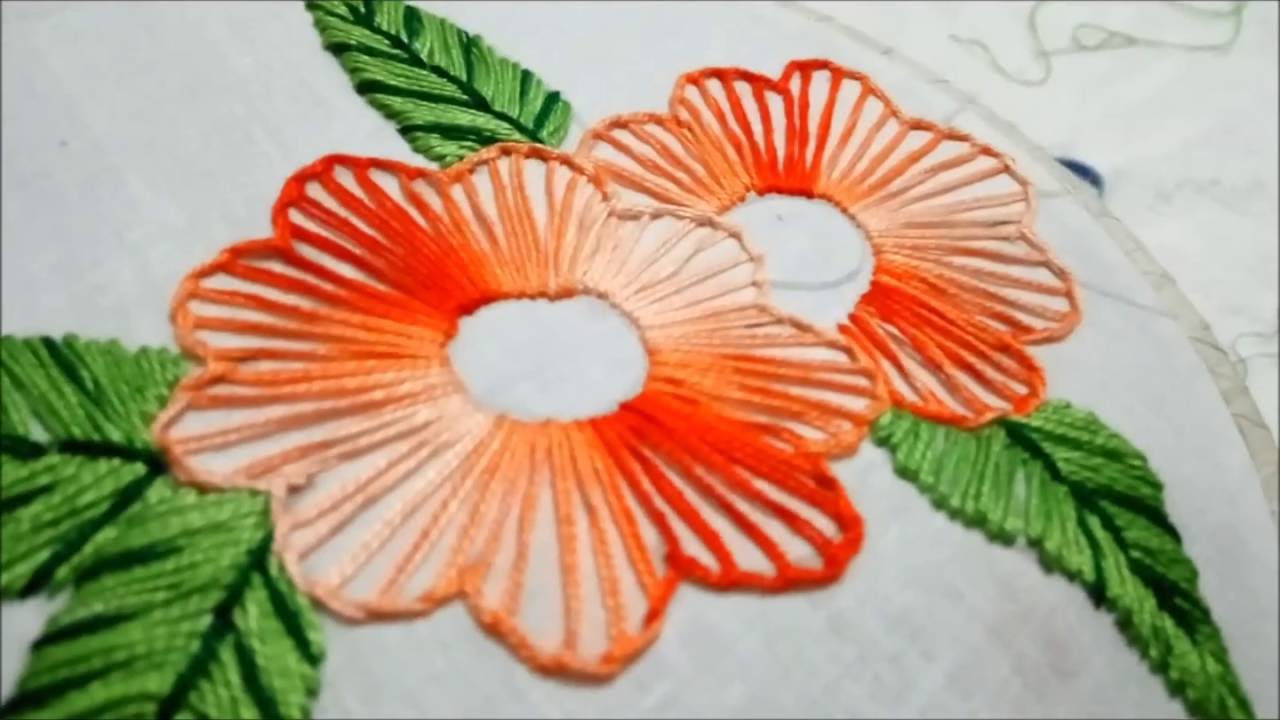The image is a detailed close-up photograph of a white fabric with intricate embroidery, framed by a thin black border. The scene is set against a whitish-gray background and features a sewing motif. Central to the composition are two prominent flowers with multiple petals, which are a blend of orange, peach, and red hues. The petals are adorned with inner stripes and are stitched in a simple, circular pattern. Surrounding the flowers are four green leaves, with two attached to each flower. Additionally, a gray stem runs from the middle right to the top. Beside the stem is a small, intricate half-circle in blue or black and a swirly stem in the upper right corner, adding to the delicate and detailed embroidery. The overall style is one of sewing and craftsmanship, highlighted by the fine details of the stitch work on the white fabric.